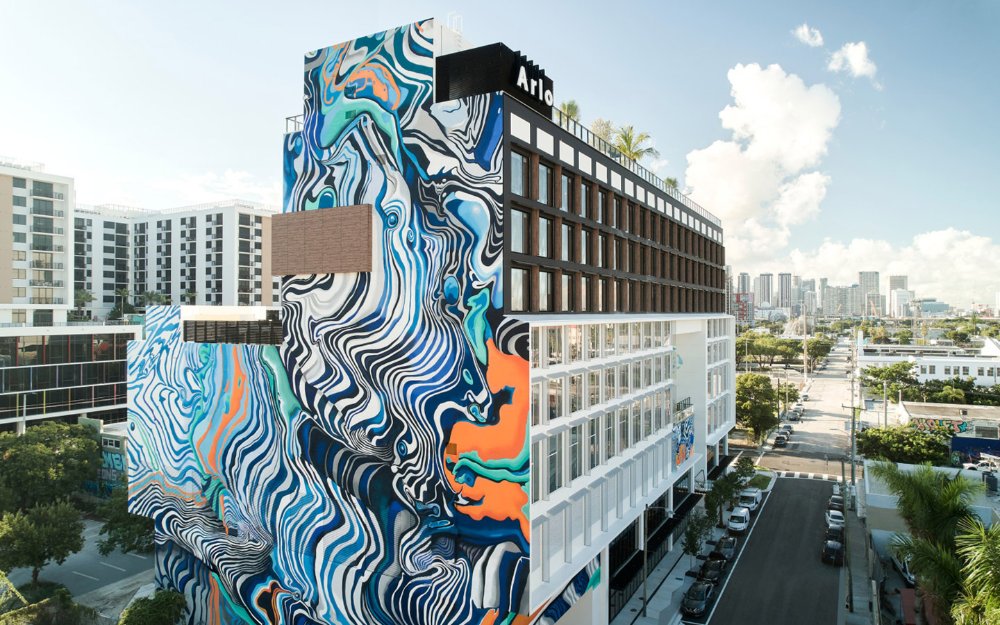This detailed photograph captures an outdoor city street scene bathed in daytime light. The focal point is a multi-story building, potentially a hotel or office space, standing prominently with the name "ARLO" displayed in white letters on a gray section at the top. The building itself rises to about eight or nine stories, featuring a structural design where the first four stories are framed in white with windows, and the subsequent four are framed in dark gray.

The most striking feature is the expansive mural that adorns one entire side of the building from top to bottom. This mural exhibits a mesmerizing array of swirling patterns and colors, including black, white, various shades of blue, along with touches of orange and green. The intricate design conjures images that are open to interpretation, such as abstract shapes or even elements resembling a lion's mouth or eyes, created through the dynamic, wavy lines.

The scene on the ground includes a bustling street with cars parked along the sides, directing the viewer’s focus toward a distant city skyline filled with towering skyscrapers. The photo also includes multi-story apartment buildings and lush trees, including palm trees, in the left and right corners of the image. The sky overhead is a pale blue, featuring scattered white clouds and a hint of thunderclouds, adding a dynamic depth to this urban composition.